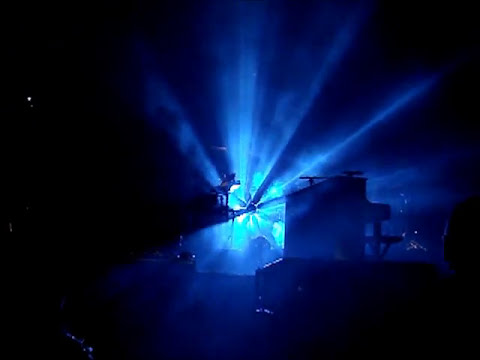The image is a square photograph depicting a dimly lit stage, dominated by black and blue hues. The left side and the upper and lower right corners of the image are enveloped in solid black. In the center, a male musician—possibly the lead singer and potentially wearing a cowboy hat—appears to be seated, perhaps strumming a guitar. The surroundings are faintly illuminated by blurry, diagonal blue spotlights or laser beams, creating an ethereal and somewhat unclear atmosphere. There is vague evidence of an instrument, likely a piano or a podium, near the musician. The stage setting suggests a large concert, with the musician highlighted prominently amidst the otherwise dark environment. Blue lights streak from the background towards the foreground, barely illuminating what could be the reflection of audience heads at the bottom. The overall scene, bathed in blue light, conveys the ambiance of a dramatic live performance.